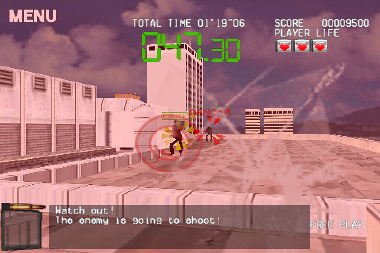The image is a screenshot of the classic arcade rail shooter, Virtua Cop, captured from a first-person perspective on the rooftop of a building. The background showcases several towering skyscrapers, providing a clear urban setting. The interface displays various game statistics: the top left corner shows the 'Menu' label, while the middle top section features 'Total Time' listed as 01:19:06 with a secondary time of 047.30 beneath it. The top right corner displays the player's score of 9500 and indicates 'Player Life' adorned with three heart icons.

At the bottom of the image, a text box warns, "Watch out, the enemy is going to shoot." This suggests imminent danger and adds a sense of urgency. The player seems to have a bullet item equipped, as indicated by the icon at the bottom right next to the 'Free Play' label. Central to the image is a red targeting reticle, composed of two concentric circles that occupy about 10-20% of the screen, aiming at multiple on-screen characters. One of these characters is actively shooting toward the player, adding to the action intensity. Another character, marked with the word 'DANGER' and surrounded by small red arrows, appears on the right side of the screen, signaling an immediate threat.

The overall visual quality of the image is pixilated, characteristic of vintage arcade games, emphasizing its nostalgic and retro feel. The detailed heads-up display, combined with the dynamic in-game action, showcases the classic arcade excitement Virtua Cop is known for.